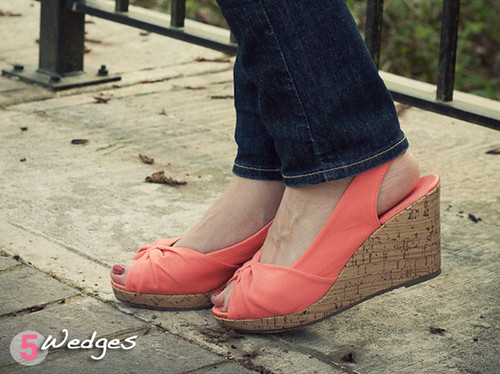This image showcases a white-skinned woman wearing dark blue jeans, standing on a grayish-tan cement sidewalk. She is modeling salmon-colored wedge sandals with fabric on the top and cork-like sides. Her toenails are painted pink. The woman is standing with her legs positioned slightly to the right, lifting one heel into the air, emphasizing the wedge shoes. In the background, a black metal railing and a green pole can be seen. Superimposed in the bottom left corner is a pink circle with the number five inside it, accompanied by the word "wedges" in white text.